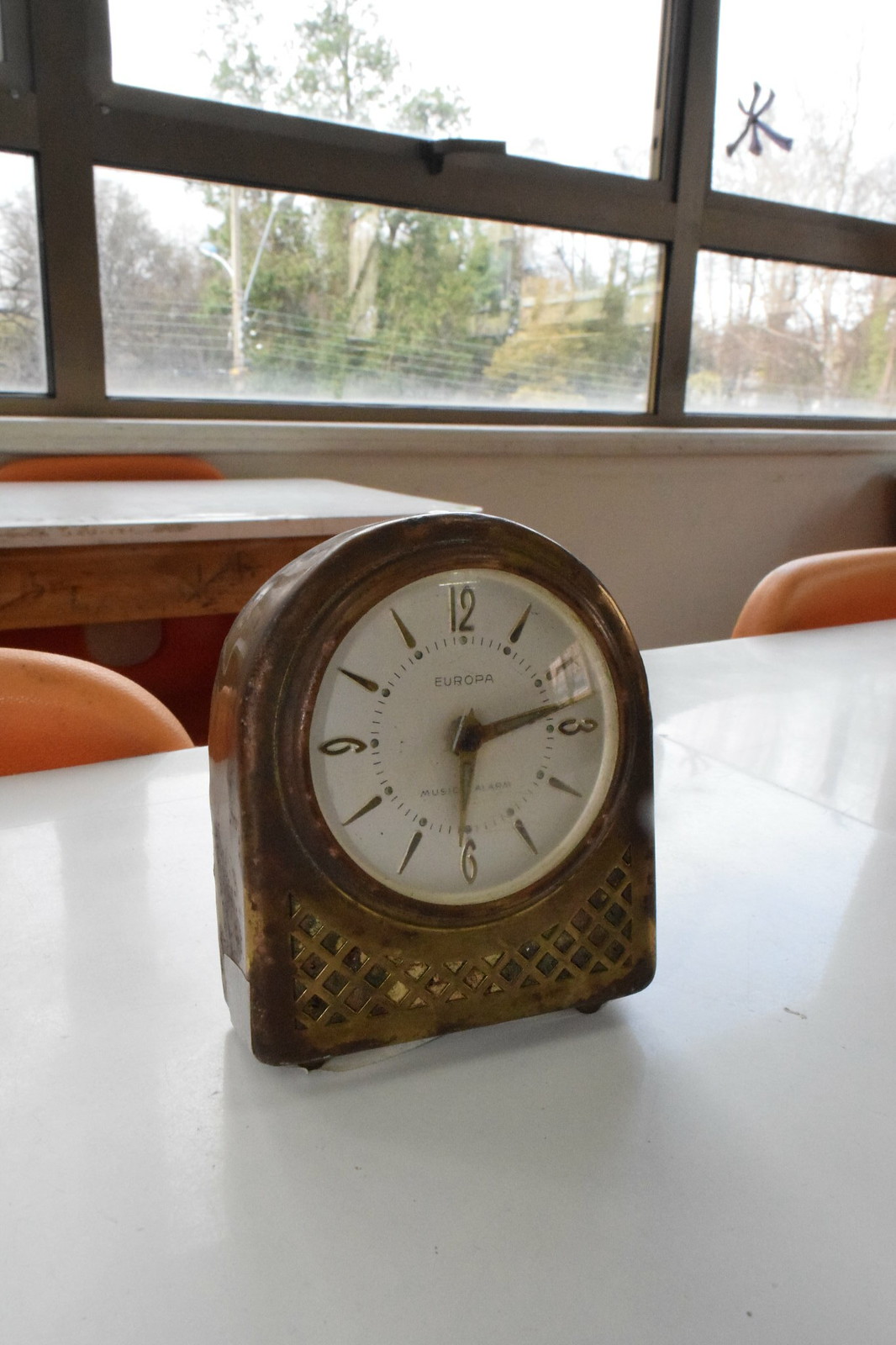The image depicts a tarnished gold mantel clock as the focal point, sitting prominently on an off-white to very light gray plastic or laminate table. Flanking the table are glimpses of two orange chairs, providing a subtle burst of color. Positioned in front of a window, the scene outside reveals trees in bloom on an overcast day, adding a touch of natural vibrancy to the indoor setting.

The clock itself features an elegant design, rounded at the top and flat at the bottom. Its white face is adorned with gold numbers, with the 12, 3, 6, and 9 numerals clearly defined, while the remaining positions are marked by small, teardrop-shaped emblems. Minute markers are meticulously placed in the form of small white circles denoting five-minute intervals, accompanied by gold or silver slashes for each minute.

Beneath the 12 o'clock position, the word "EUROPA" is prominently displayed in uppercase letters. The clock hands, also gold, are finely pointed, with the minute hand slightly longer than the hour hand. The time reads just past 6:13. Below the clock face, a mesh design stretches from end to end, adding a layer of texture. The clock stands firmly on two small visible feet, possibly supported by two additional feet at the back, completing its solid yet intricate structure.